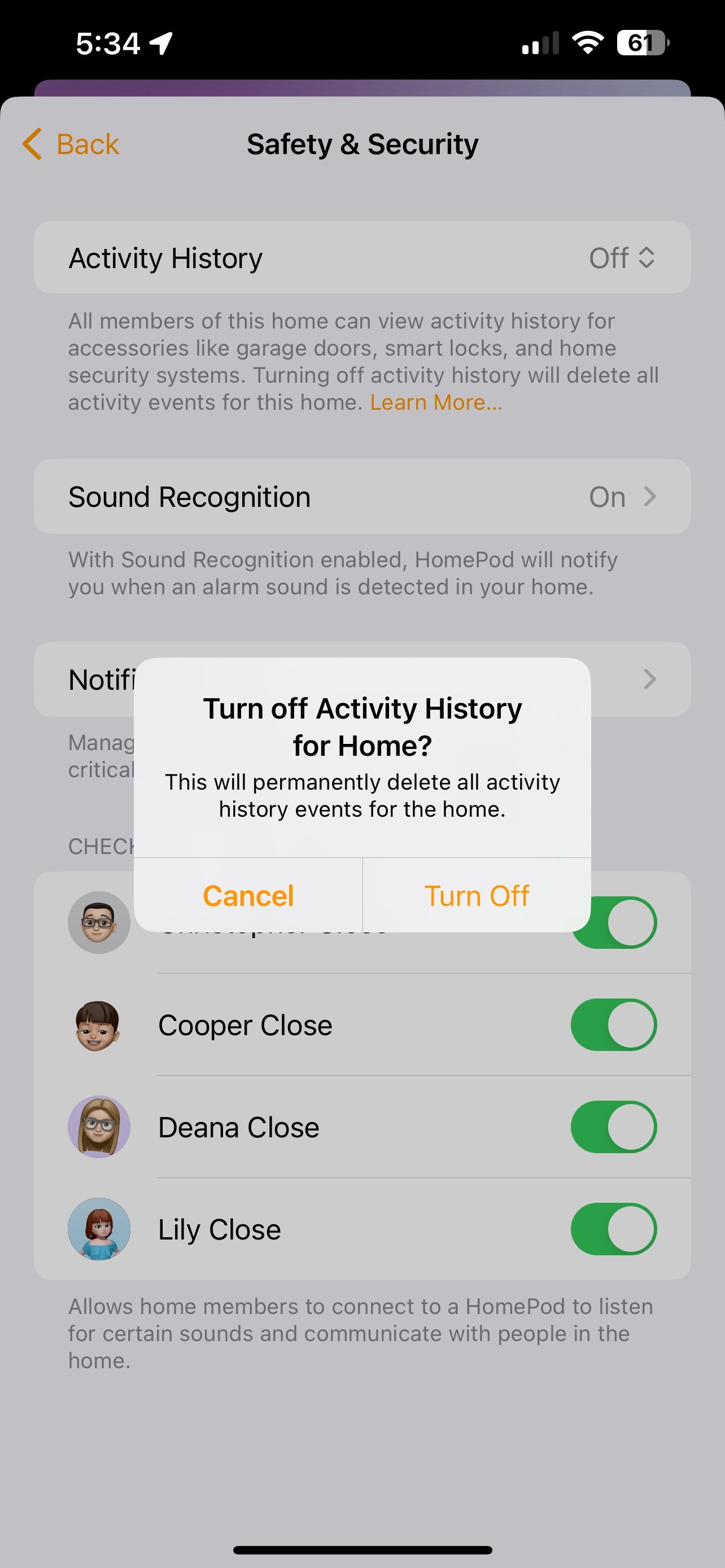This image, captured in portrait format from a mobile phone, showcases the "Safety and Security" settings of a home security application. The screenshot's top border features a black strip with crucial mobile indicators: the time displayed at 5:34 am, an arrow icon pointing northeast, and three status icons to the right displaying partial signal strength, WiFi connectivity, and a battery level at 61%.

The main content begins with the "Safety and Security" header in bold. On the left, an orange "Back" text is accompanied by a back arrow. Below this, a grey banner spans the width of the screen, stating "Activity History" on the left and "Off" with an up-down arrow on the right. Beneath this banner, informative text explains that activity history lets all family members view actions related to smart home accessories such as garage doors, smart locks, and security systems, and turning off this feature will delete all recorded events. An orange "Learn more..." text prompt concludes this section.

Further down, another grey banner indicates "Sound Recognition," showing "On" with a right arrow on the right. The accompanying text reveals that enabling this feature allows the HomePod to notify the user upon detecting alarm sounds within the home.

The next section, partially obscured by a pop-up, starts with a grey banner labeled "Notification," truncated to "Notify" on the left, with a right arrow on the right. The white pop-up message dominating the center of the screen reads, "Turn off activity history for home? This will permanently delete all activity history events for the home." At the pop-up's bottom, "Cancel" is displayed in bold orange, while "Turn off" is slightly less prominent to the right.

Underneath this notification, visibility is limited due to the pop-up. However, it appears to feature face avatars in a grey box with accompanying names and toggle buttons. Notably visible avatars include a young Caucasian male named Cooper Close, a young Caucasian female named Diana Close, and another labeled Lily Close wearing a blue dress, all with active green toggle buttons on the right. The section concludes with text explaining the purpose of allowing home members to connect to the HomePod for sound notifications and communication.

Overall, the image provides a detailed glimpse into the "Safety and Security" settings of a home security app, juxtaposed by a central pop-up notification prompting the user to confirm or cancel the deletion of activity history. The backdrop dims slightly, highlighting the pop-up as the focal point.